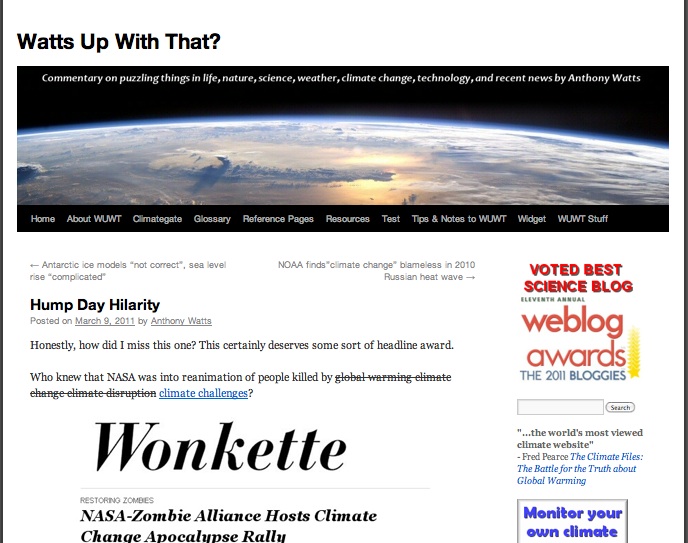This image showcases an article topped with the headline, "What's Up With That?". Below the headline, there is a striking picture of space, featuring clouds illuminated by distant lights and a distinct border of darkness enveloping part of the scene. Surrounding this picture, the text points to a community focused on puzzling aspects of life, nature, science, weather, climate change, technology, and recent news, curated by Anthony Watts. Below the picture, there is a navigation bar with sections like Home, About WJWT, Climate Change Documentary, Reference Pages, Resources, Tests, Tips, and Nature. At the article’s end, the text reads, "Hump Day Hilarity: Honestly, how did I miss this one? This certainly deserves some sort of headless award, I think." The closing lines continue, "Who knew NASA was into re-ermination people killed by global warming, climate change?" concluding this curious piece.